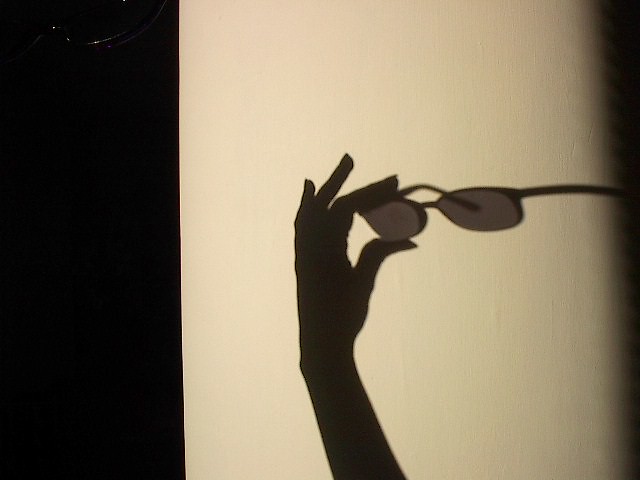The image is a realistic photograph, primarily in black and white, formatted as a horizontal rectangle. The left quarter of the image is dominated by a black horizontal rectangle, creating a stark contrast with the rest of the picture. Toward the center of the image, there is a light beige or slightly off-white vertical surface, likely a wall, illuminated in such a way that it appears somewhat yellowish. Near the middle of the image, a clear shadow outlines a left hand with long, thin fingers and potentially manicured nails, suggesting it might be a woman's hand. The shadow depicts the hand from the wrist up, with the thumb and index finger holding a pair of sunglasses by the nose piece. The sunglasses, fully extended with both lenses and ear pieces visible, are silhouetted crisply against the lit background. On the right side of the image, more shadows and darkness frame the focal hand and sunglasses, adding depth to the composition. No additional text or elements are present in the photograph, keeping the focus on the play of light and shadow.